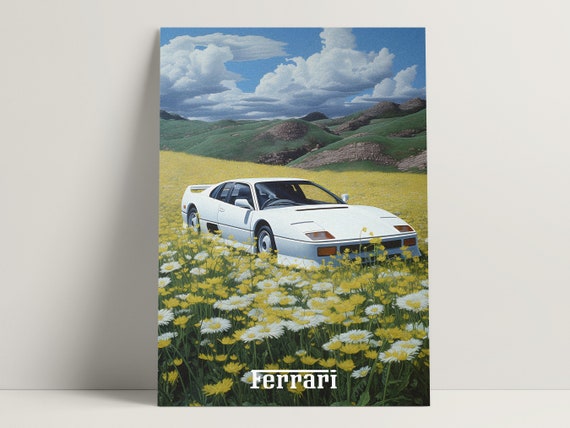The image is a detailed poster of a white Ferrari sports car leaning against a white wall and resting on a white surface. The poster itself features a beautiful landscape with the Ferrari parked in a sprawling field filled with daisies, predominantly yellow, with some white ones mixed in. The vibrant field extends towards green rolling hills peppered with gray and brown rocks in the background. The sky above showcases a brilliant blue hue, dotted with large, fluffy white and gray clouds, and although the sun is not visible, its light illuminates the scene effectively from behind the car. The Ferrari, equipped with a spoiler, orange and clear headlights, and black tires with white rims, sits prominently in the serene, sunny field, with "Ferrari" inscribed in white text at the bottom center of the poster. The composition and lighting suggest a naturally moderate brightness without professional enhancements, while the car and scenery stand out vividly against the plain white background of the setting.